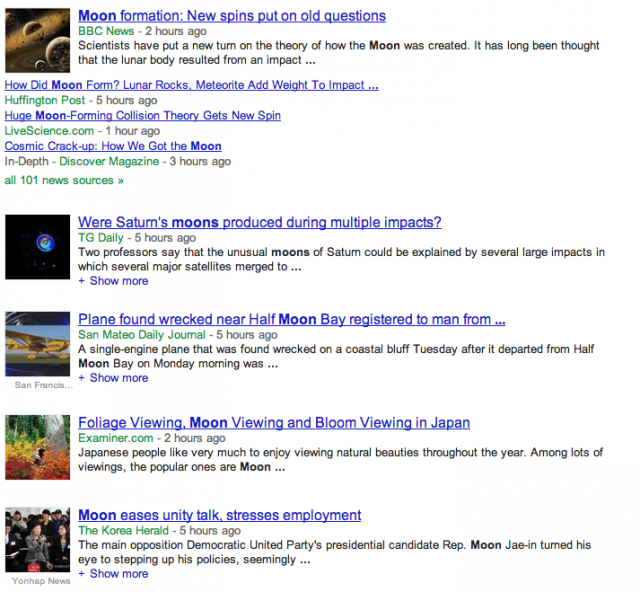Descriptive Caption:

The image displays search results from a search engine, showcasing recent news articles about lunar formation theories. At the top, an article from BBC News titled "Moon Formation: New Spins Put on Old Questions" discusses how scientists have introduced a new perspective on the moon's creation, historically believed to result from a colossal impact. Accompanying this headline is an icon depicting moons.

Below, several other articles are listed. One from LiveScience.com, titled "How Did Moon Form? Lunar Rocks, Meteorite Add Weight to Impact," highlights new evidence supporting the impact theory. Another, "A Huge Moon Forming Collision Theory Gets New Spin," delves into the evolving understanding of the moon's origins. 

Additionally, an article from In Depth titled "A Cosmic Crack Up: How We Got the Moon" is featured, each entry showing their respective publication dates.

Further down, a series of thumbnails and article headlines appear. These include topics like Saturn's moons, a plane wreck found near Half Moon Bay, and cultural activities in Japan such as foliage and moon viewing. Another headline discusses unity and employment in relation to the moon.

Each article is accompanied by a small image to the left, enhancing the visual appeal of the search results.